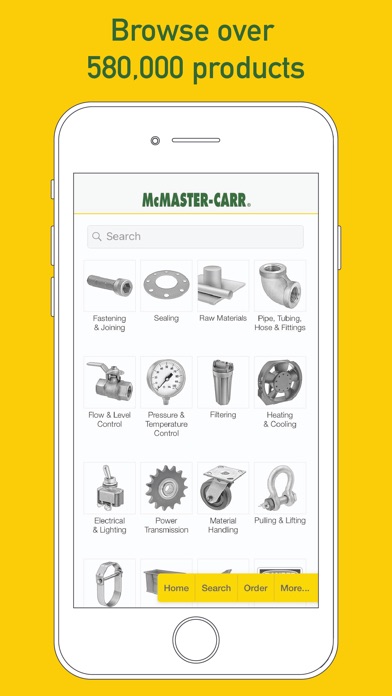The vertical image features a bright yellow background with prominent, olive green text at the top that reads "Browse over 580,000 products" in two lines. Below the text is a simple illustration of a smartphone's front view. At the top of the smartphone's screen is a vertically oriented box outlined in grey, displaying "McMASTER-CAR" in green, capital letters. A thin yellow line separates this header from a search bar beneath it.

Further down, the image showcases a grid with four rows of four icons each, representing different product categories. Each icon is a simple drawing accompanied by text. The categories in the first row are: "Fastening and Joining," "Sealing," "Raw Materials," and "Pipe, Tubing, Hose, and Fittings." The second row includes: "Flow and Level Control," "Pressure and Temperature Control," "Filtering," and "Heating and Cooling." The third row lists: "Electrical and Lighting," "Power Transmission," "Material Handling," and "Pulling and Lifting." Notably, the bottom-left icon is blank.

Covering the bottom three icons is a thin yellow bar with four buttons labeled "Home," "Search," "Order," and "More." Additionally, a large circle at the bottom of the smartphone represents the device's physical home button.